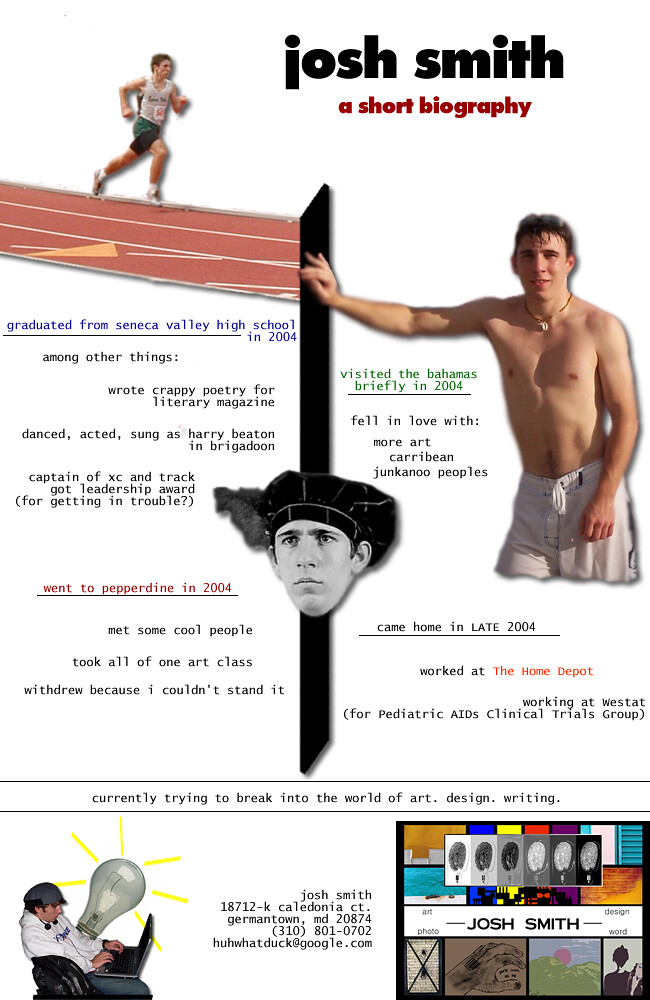The image is a detailed, visually colorful biography of Josh Smith set against a white background. At the top right, it prominently displays the name "Josh Smith" in black text, followed by "a short biography" in smaller red text. On the upper left, a photo shows Josh in a track suit running on a racing track. Below it, blue text reads "Graduated from Seneca Valley High School in 2004." The biography continues in black, noting his various activities, including writing poetry for the Literary Magazine, dancing, acting, singing as Harry Beaton in "Brigadoon," serving as the captain of the cross-country and track team, and earning a leadership award for his troublemaking.

A black line runs vertically down the center of the page, featuring a black-and-white portrait of Josh wearing a large black cap. On the right side, a shirtless Josh in white shorts leans against this black bar. Green text notes that he "visited the Bahamas briefly in 2004," and black text follows, saying he "fell in love with more art, Caribbean culture, and the Junkanoo people." It continues to describe how he returned home in late 2004 and worked at both The Home Depot and Westat for the Pediatric AIDS Clinical Trials Group.

In black text, it also states, "Currently trying to break into the world of art, design, and writing." Below left, there's another image of Josh using a laptop with a light bulb graphic, while to the lower right, personal details including his contact information, "John Smith, 18712K, Caledona Court, Germantown MD 20874, 310-801-0702," along with an email address, "Oh, what a duck at google.com," are provided. A webpage capture and a small graphic of various items further embellish the right side.